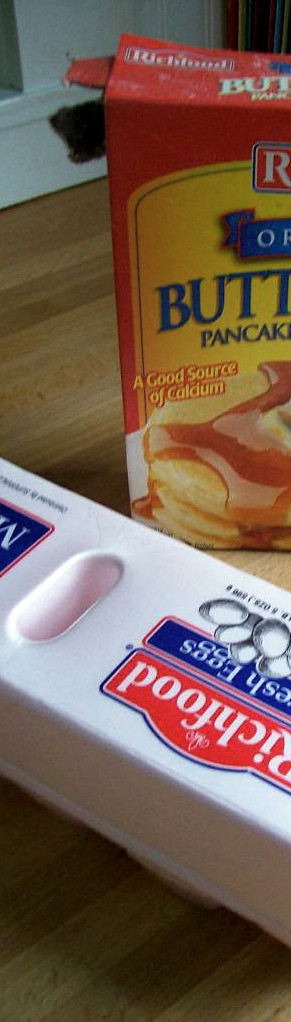In this image, a white egg carton labeled "Rich Food" prominently features a bright red label. Above this label is a blue patch with the words "Fresh Eggs." The carton is adorned with illustrations of eggs. Resting on top of the egg carton is a red box of pancake batter, which is accented with yellow coloring and boasts that it is a good source of calcium. Both items are situated on a brownish wooden surface, which could either be a tabletop or hardwood flooring. In the background, a white wall can be seen, and notably, the pancake batter box appears to have been opened along the side.